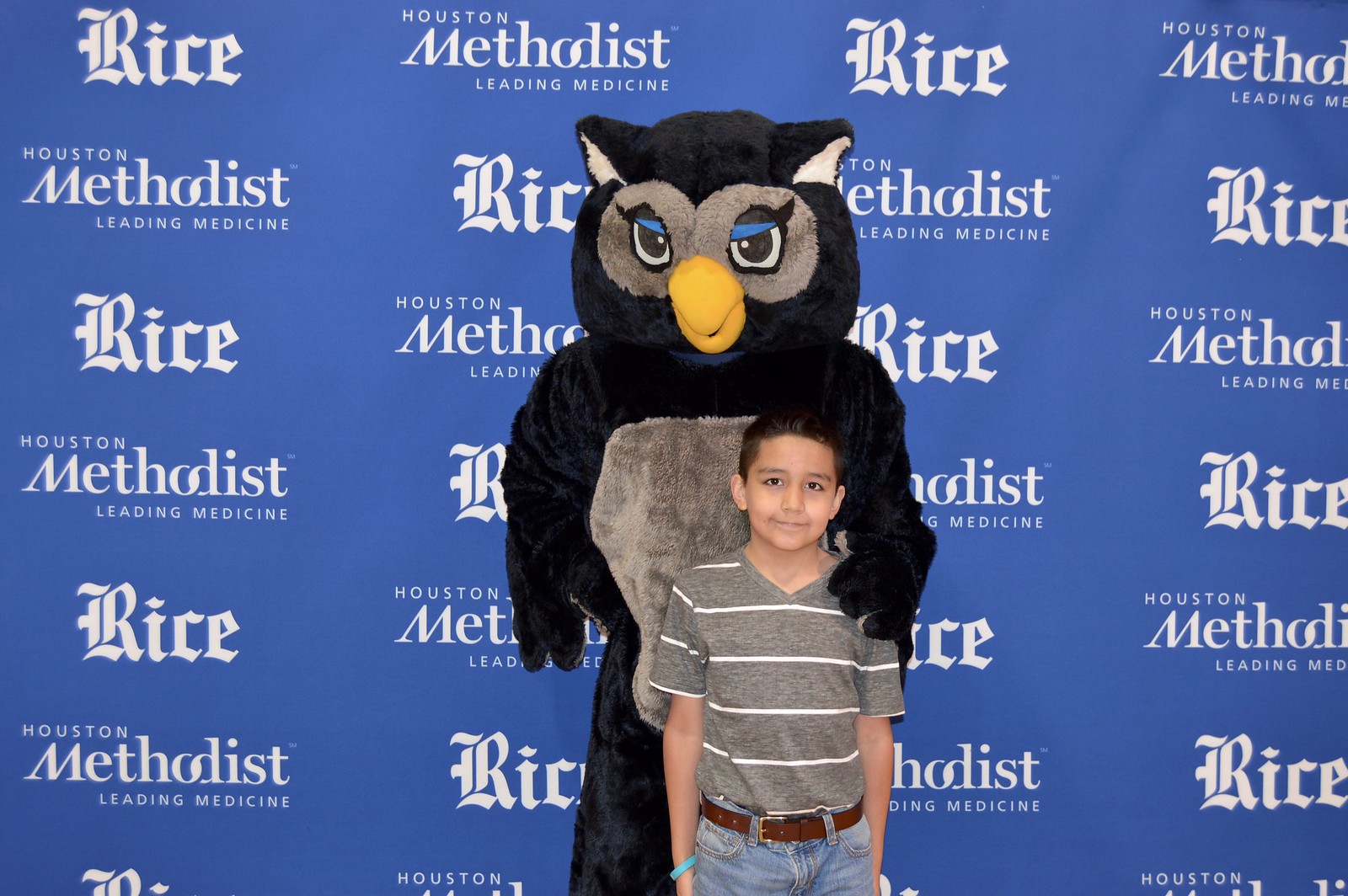In the image, a young boy with short black hair and light brown skin is posing in front of a blue backdrop adorned with white logos reading "Houston Methodist Leading Medicine" and "Rice." The boy is dressed in a gray V-neck t-shirt with thin white stripes, blue jeans, and a brown belt. Behind him stands a large mascot, an owl with a deep navy blue fur body, a gray belly, and distinguishing features such as blue eyelids over its big black eyes, a yellow beak, and white insides on its ears. The owl mascot has its hand resting gently on the boy's right shoulder, adding a friendly and protective presence to the photograph.